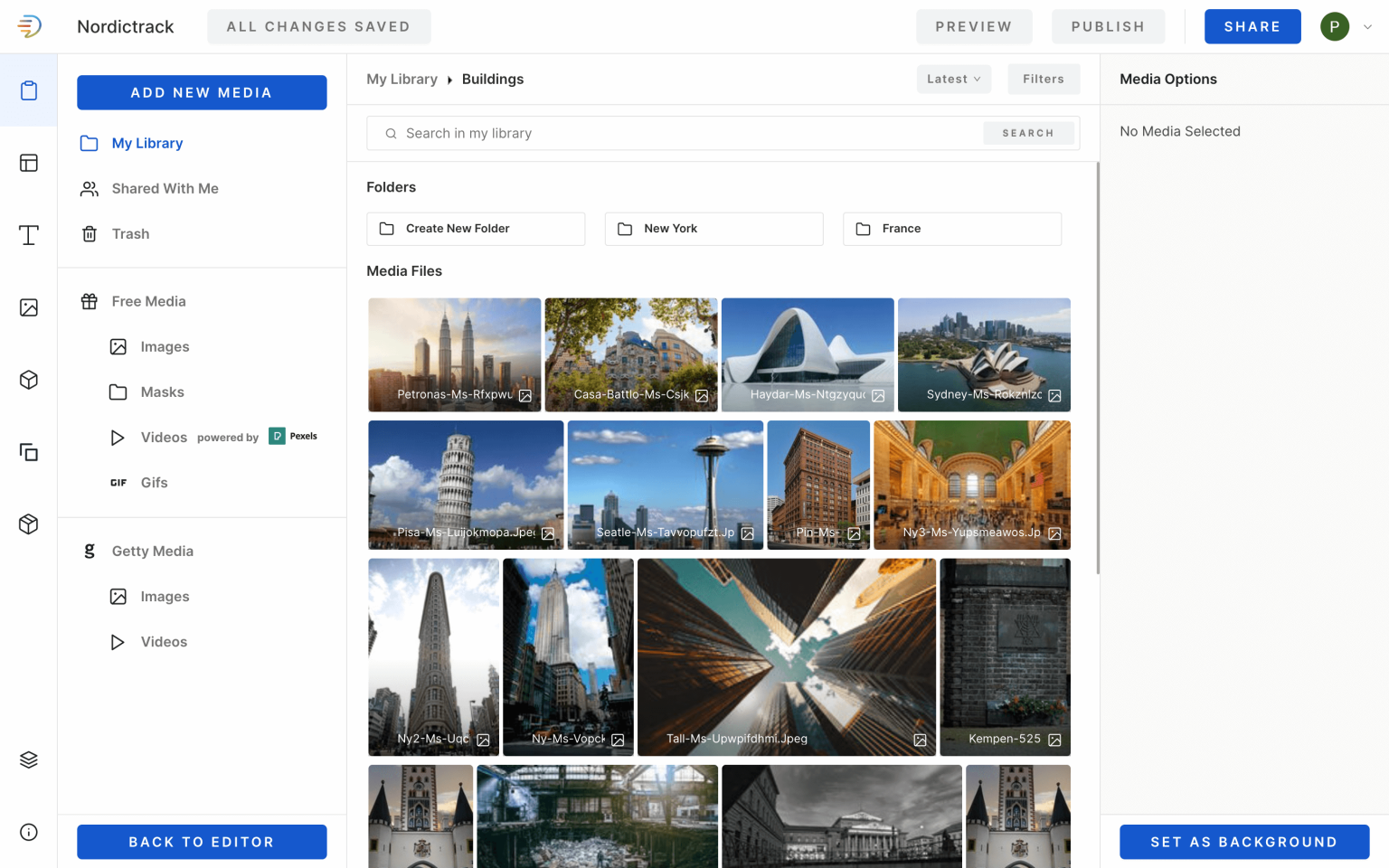The web page displayed is from NordicTrack, featuring a comprehensive left navigation pane. This sidebar includes various options such as "Add New Media," "My Library," "Shared With Me," "Trash," and "Free Media." In terms of media types, the user can choose from "Images," "Masks," "Videos Powered by Pexels," and "GIFs." Additional navigation items allow the user to manage their media with options like "Get to Media," "Images," "Videos," and "Back to Editor."

Within "My Library," there are categories like "Buildings," and a search bar labeled "Search in My Library." Users can also organize media in "Folders" or create a new folder. Among the listed folders and media files, specific labels include "New York," "France," "Petronas," "Pisa," "New York 2," "Seattle," "Seoul," and "Campaign 5 to 5."

Overall, the interface is designed to help users efficiently manage various types of media with an easily navigable and organized layout.